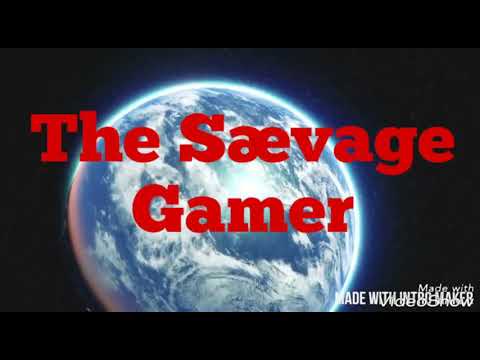This digitally created horizontal image features the Earth from space set against the black void of outer space with darker black borders on the top and bottom. The Earth, depicted in a blend of blue oceans and white cloud covers, dominates the foreground, though individual continents aren't discernible. Prominently displayed across the image in bright red font are the words "The Saevage Gamer," with "Saevage" notably misspelled as S-A-E-V-A-G-E, including a ligature combining 'A' and 'E'. In the lower right-hand corner, overlaid text in white font attempts to state "Made With Intro Maker," obscured by overlapping elements that render it partially illegible. The composite nature and overlays suggest the image might be a screen capture from a video or a digital advertisement for a gaming system or game, rather than a standalone photograph.